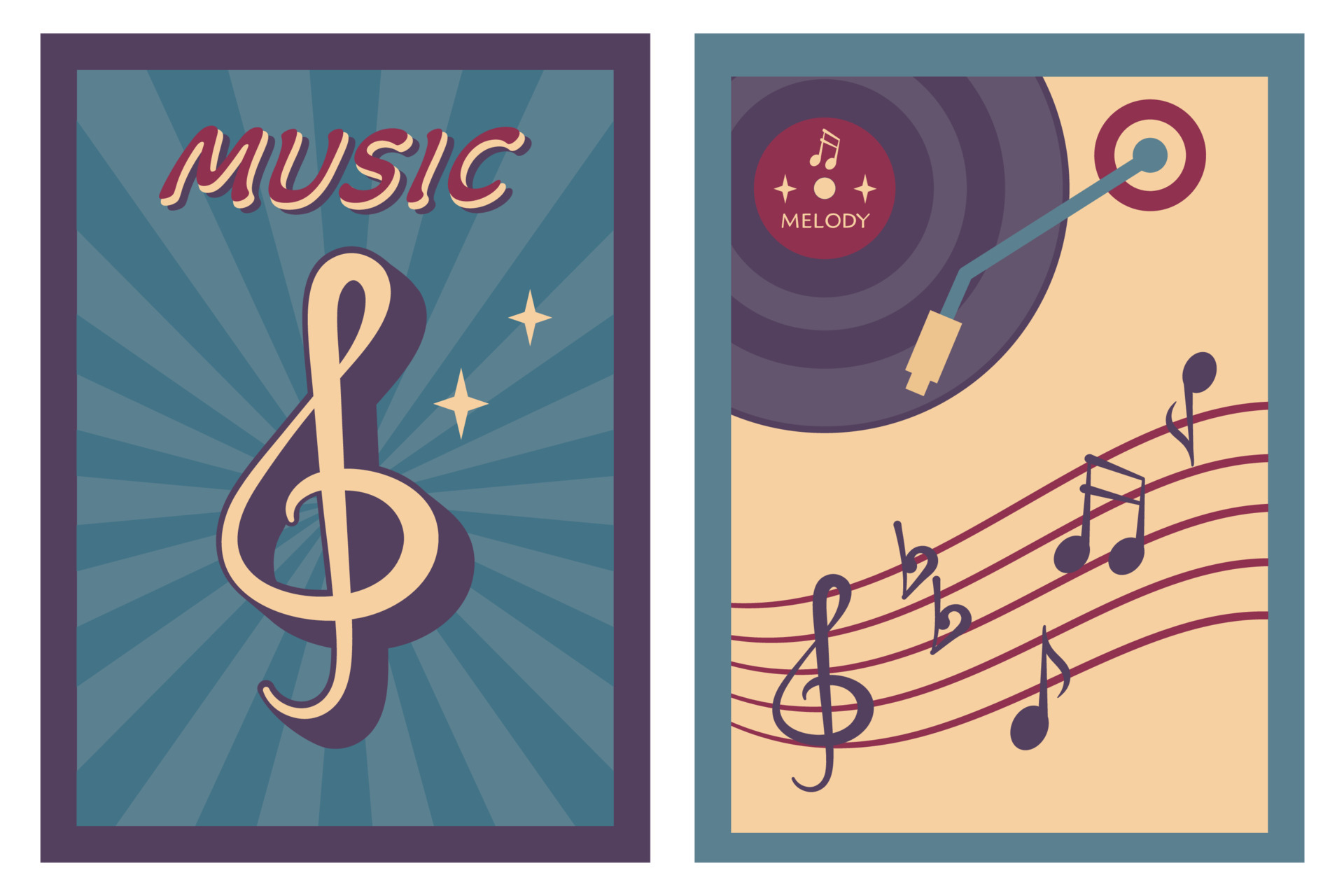The image features two flat, non-three-dimensional, computer-generated posters with a distinct pop art style. Both posters display a striking palette of blue, turquoise, purple, beige, and red tones.

**Poster on the Left:** Framed with a dark purple border, the poster showcases the word "MUSIC" in bold, reddish-purple capital letters with cream-white highlights. Below the text, a dark purple treble clef symbol is set against a vibrant blue and light blue sunburst background. Two small white stars add a touch of sparkle adjacent to the clef, enhancing the dynamic feel of the design.

**Poster on the Right:** Enclosed in a blue border with a beige background, this poster features a vintage vinyl record in the top left corner. The record is rendered in purple tones with light purple stripes and a reddish-purple center. The word "MELODY" is inscribed on the record. Below the record, a series of musical notes and a treble clef float across the bottom, outlined in light blue, adding a rhythmic flow to the composition.

Both posters are characterized by their flat, illustrative style, reminiscent of old Western cartoon images, blending modern graphic design elements with nostalgic motifs.